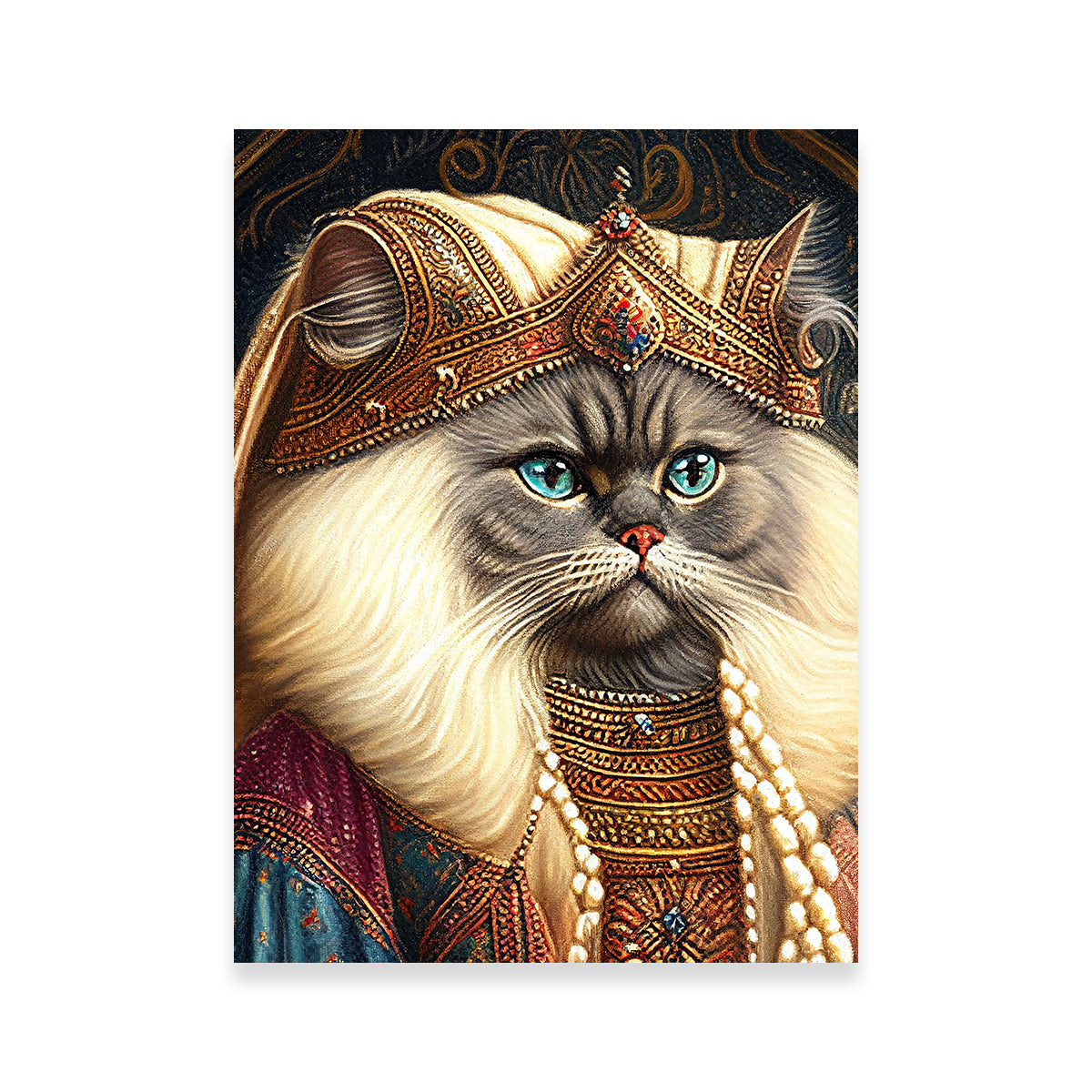This detailed art drawing features a majestic gray cat with long, flowing white hair accentuating its face. The cat, boasting light blue eyes and a distinctive red nose, holds an air of royalty with its white whiskers and ornate ensemble. It wears a unique crown, possibly made of leather or cloth, adorned with intricate designs and an array of jewels in blue and red. The crown is gold with maroon hints and features a prominent teardrop-shaped jewel at the front. The cat is also dressed in a resplendent cloak or vest, a blend of gold, magenta, and blue hues, embellished with various gems. This attire, combined with its upright, regal posture, gives the impression of feline royalty. The overall composition might evoke thoughts of ancient civilizations like Egypt, where cats were revered. The cat gazes directly ahead with its striking light blue eyes, merging human-like sophistication with its natural elegance.